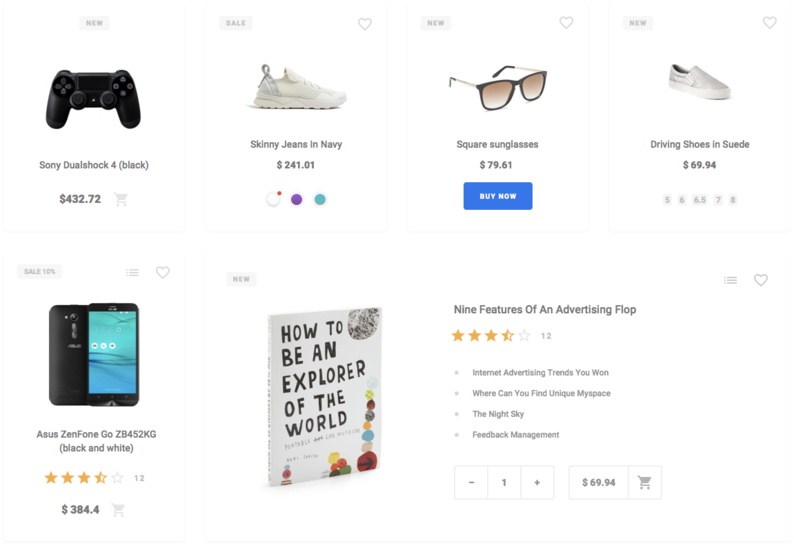A detailed screenshot of an initial visit to a sales page showcases several seemingly mismatched product listings. On the top left corner, there is a listing for a Sony DualShock 4 controller in black, oddly priced at $432.72. Adjacent to it, a listing for "navy skinny jeans" features an image of a white tennis shoe priced at $241.01. Beneath this, there's a product labeled "square sunglasses" for $79.61, but the image displayed shows sunglasses that are rounded and rectangular. Next to the sunglasses, a listing for "driving shoes in suede" shows slip-on skating shoes instead, priced at $69.94. On the bottom left of the second row, an Asus Zenfone Go ZB452KG in black and white is listed with a 4-star rating for $384.40. Finally, there is a book titled "How to Be an Explorer of the World: 9 Features of an Adventure Flop," also rated 4 stars and priced similarly to the shoes, at $69.94.